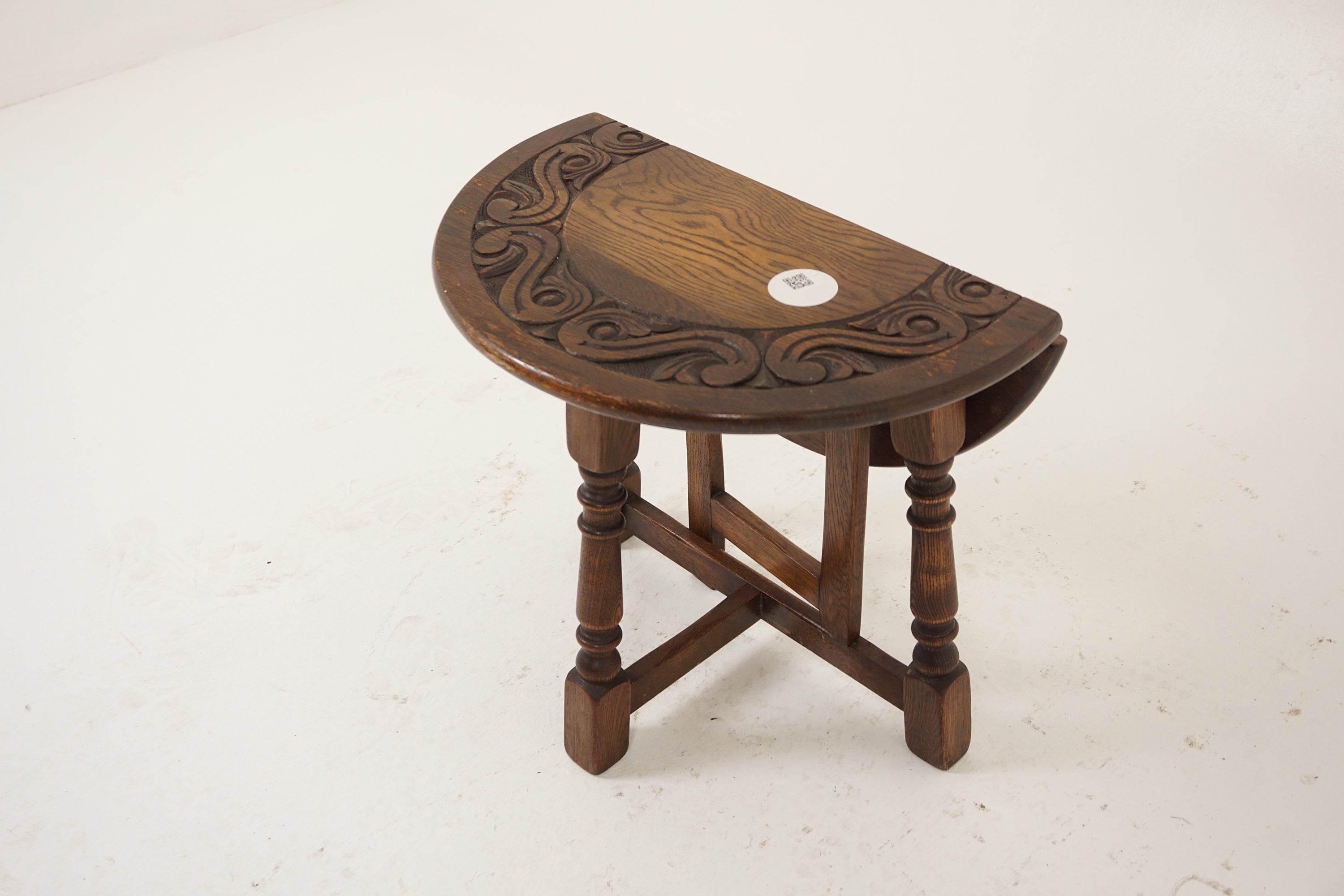The image depicts an antique-style folding wooden table designed to transform between a coffee table and a study desk. The table features a rich brown finish with a distinctive wooden grain and ornate carvings, including an intricate filigree pattern that extends in an arc around a central circular wood grain detail. The surface shows signs of wear and erosion, indicative of its age, and bears a circular white sticker with a QR code in the center. The table’s design includes a unique three-legged structure with an H-shaped wooden frame that supports a section of the table that folds down. This modular design allows the table to be used as a full circle or folded into a half-table configuration, which can be conveniently placed against a wall. The table captures the viewer's focus as it sits centrally in the image, against a beige background and a white floor marked with scratches and dirt, suggesting a well-used piece of furniture possibly of Danish origin and potentially around 100 years old.